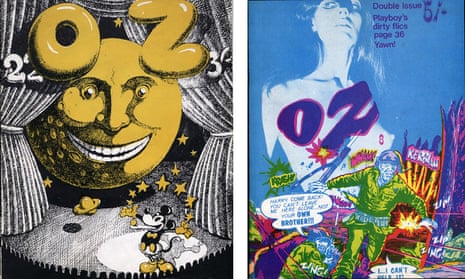This artwork features two distinct posters side by side. The left poster, rendered mostly in black and white with hints of dark mustard yellow, depicts a stage scene. At the center is an old-time Mickey Mouse, reminiscent of the Steamboat Willie era, juggling several gold stars. Perched on the floor is a small golden planet Saturn. Overseeing this scene is a deviously smiling moon, or possibly a sun, peeking through parted black and white curtains at the back of the stage. Above the moon are the letters "OZ" in a balloon-like golden font. The numbers "22" and "39" are also visible on the stage curtains.

The right poster is dominated by a blue background and features a large, purple "Oz" at the top. Below this, a Caucasian woman with long hair gazes upward and to the side. Her one exposed breast and the words "Double Issue," "Playboys," "Dirty Pics," "Page 36," and "Yawn!" are scattered around her form. Additionally, a comic-style scene is depicted at the bottom, showing a green-uniformed soldier with a blue helmet running out of an explosion rendered in shades of red, yellow, and orange, while another soldier ducks nearby. Surrounding the soldiers are comic strip speech bubbles, although the text is unreadable.